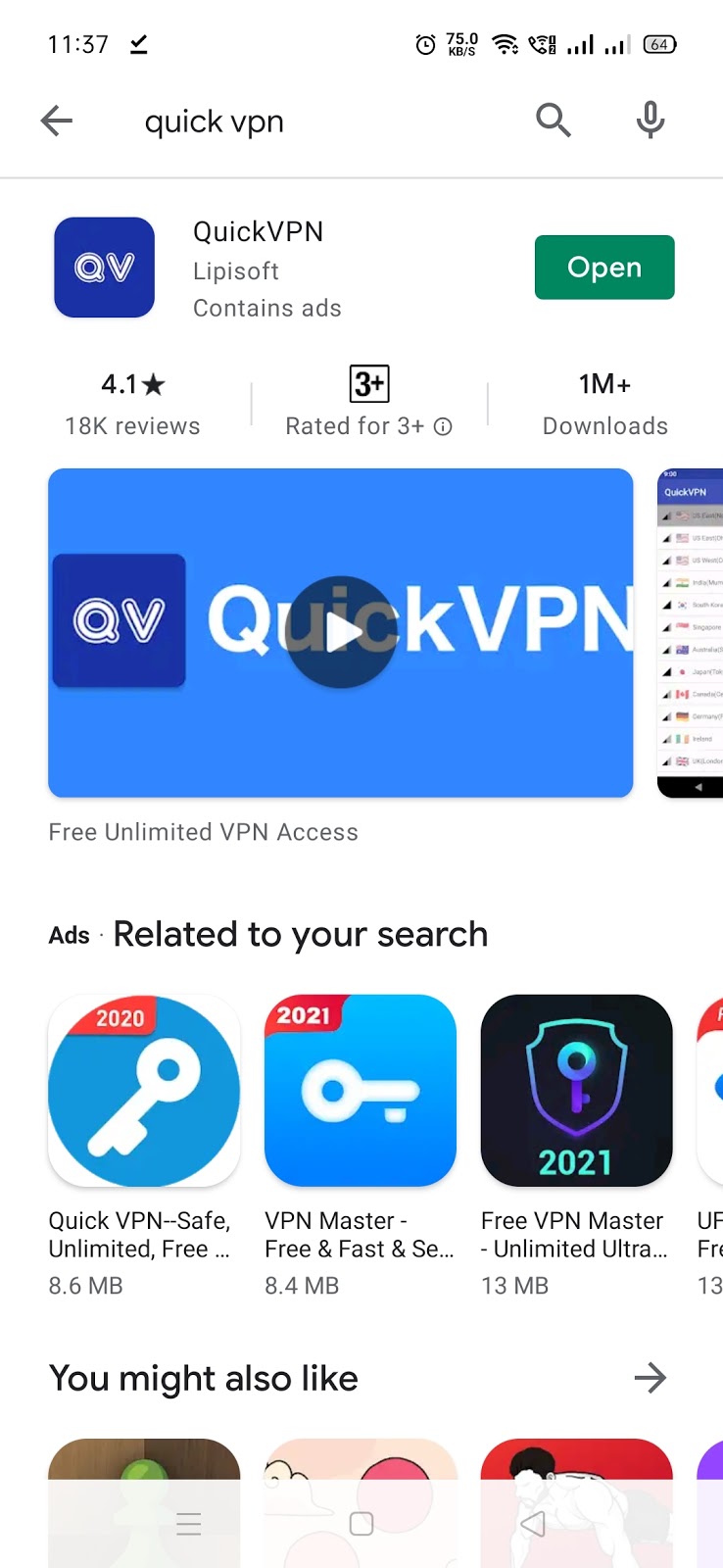The image depicts the Google Play Store interface with a search bar located at the top left, where the text "Quick VPN" has been entered. Below the search bar, the first search result displayed is an app named "Quick VPN" by Lippisoft. To the left of the app name is the app icon, which features a blue background with "QV" written in white.

To the right of the app name is a green button with the text "Open" written in white. Underneath the app name, the app has a rating of 4.1 stars out of 5 based on 18k reviews. Adjacent to the reviews, it specifies that the app is "Rated for everyone." Further to the right, the app has over 1 million downloads.

Below this section is a paused video showcasing the application, which includes a transparent black play button overlaying it. The background of the video frame is blue, with the app icon prominently displayed. Beneath the icon, white text reads "Quick VPN," followed by the subtitle "Free unlimited VPN access."

At the bottom part of the interface, there are advertisements labeled "Related to your search," featuring apps that are similar to Quick VPN. The ads display various VPN apps including "Quick VPN Safe Free Unlimited" and "VPN Master: Free and Fast," both of which have blue and white themes. The first app is from 2020, and the second from 2021. Additionally, there is "Free VPN Master Unlimited Ultra," characterized by a black and slightly green color scheme. The background of this advertisement section is white.

Overall, the image gives a snapshot of the Google Play Store's interface when searching for VPN applications, prominently featuring the Quick VPN app by Lippisoft and related VPN app suggestions.